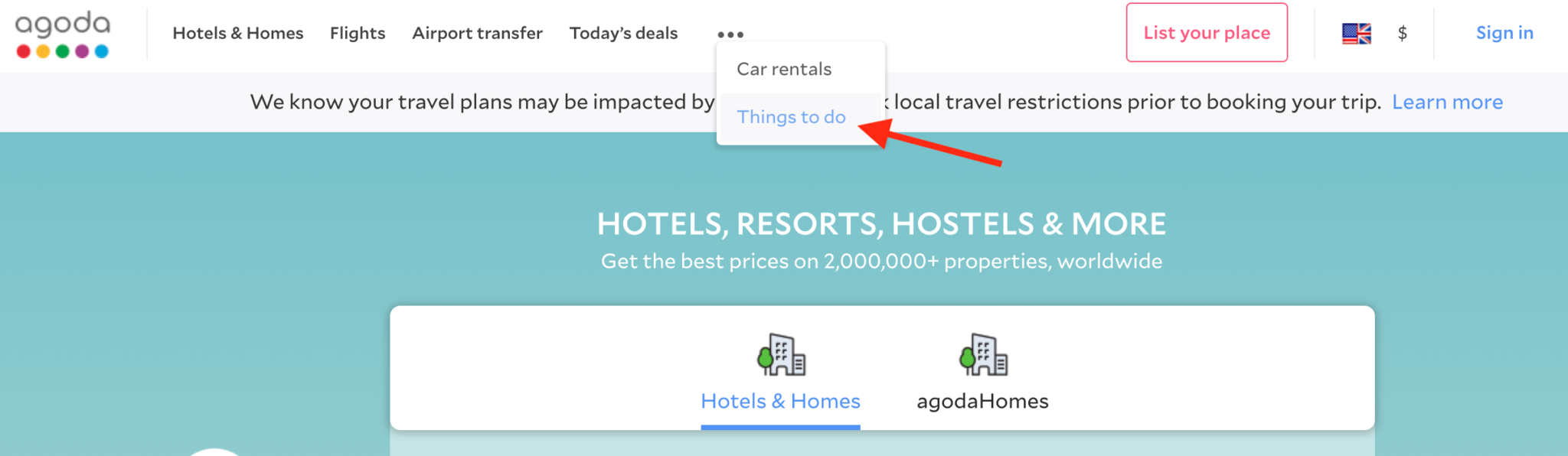**Website Navigation Bar Explained in Detail**

The image depicts a website's navigation bar, starting from the left side with the text "Hotels and Homes." Moving towards the right, the following options are listed sequentially: "Flights," "Airport Transfers," "Today's Deals," and then an ellipsis ("..."). When this menu is expanded, additional options appear, including "Car Rentals" and "Things to Do." A red arrow, seemingly added via a photo editor, points specifically at "Things to Do."

Continuing along the same navigation line, the next item is "List Your Place," which is highlighted with a red outline and features red text on a white button. Adjacent to this is a symbol combining a dollar sign and what appears to be a blend of the English and American flags, though its meaning is unclear. Further right, the "Sign In" button is displayed in blue text.

Below the navigation bar, a notification area indicates, "We know your travel plans may be impacted by," but the rest of the message is obscured by a dropdown menu. The visible part continues with "local travel restrictions prior to booking your trip. Learn more."

Further down, the text reads, "Hotels, Resorts, Hostels and More – Get the Best Price on 2 Million+ Properties Worldwide." Beneath this, a specific category is highlighted: "Hotels and Homes" is in blue, while "Agoda Homes" is in black, with a blue line underlining the text, indicating the active section of the website.

The background for the "Hotels, Resorts, Hostels and More" section is a medium turquoise blue, featuring white font, while the rest of the website has a white background with black text.